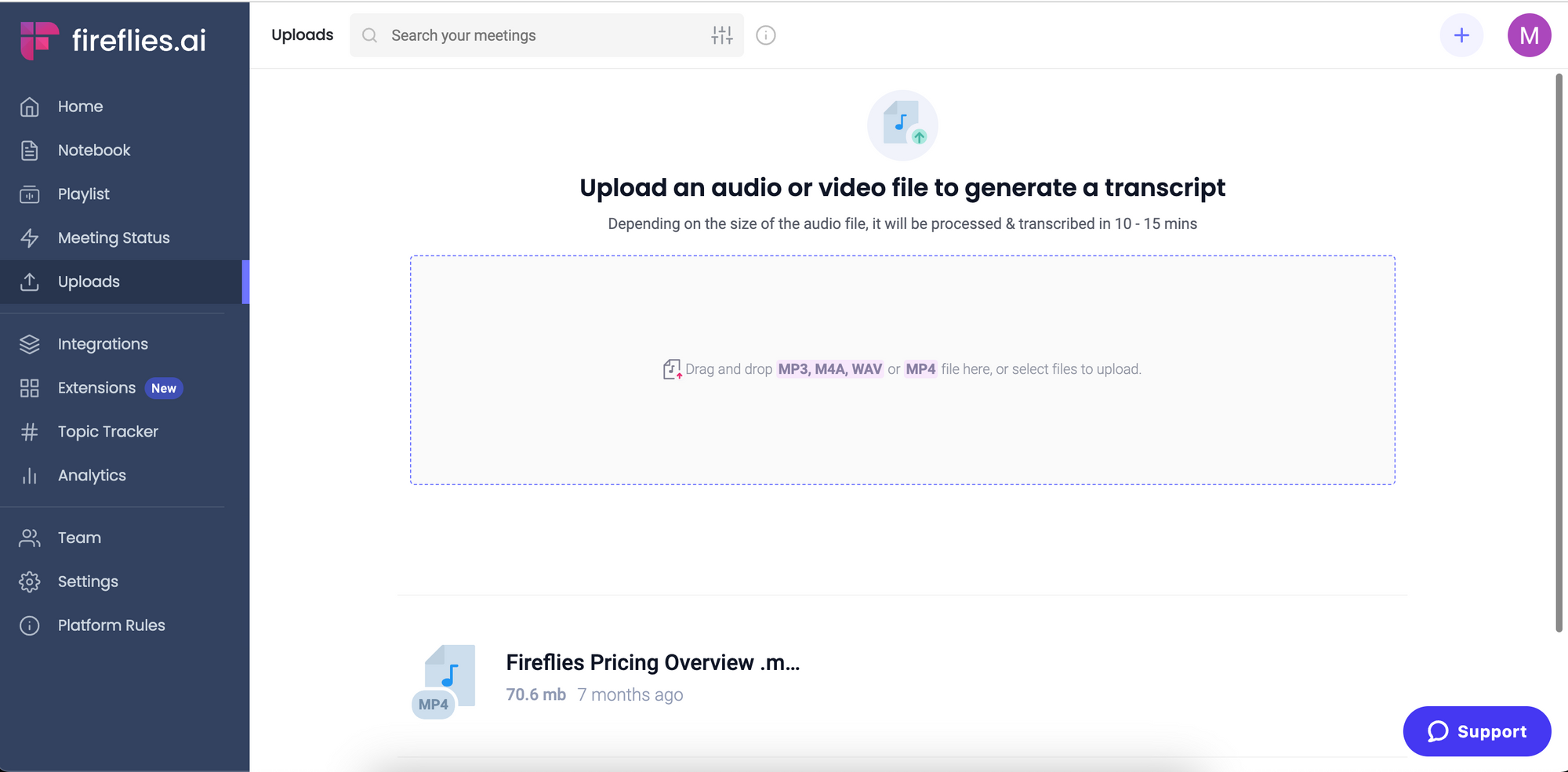The screenshot, taken from the Fireflies.ai platform, features a detailed interface layout. In the top left corner, the Fireflies.ai logo is visible. A dark navy sidebar displays various navigation buttons including: Home, Notebook, Playlist, Meetings, Status, Uploads (highlighted as currently selected), Integrations, Extensions (marked as new), Topic Tracker, Analytics, Team, Settings, and Platform Rules.

On the right, a modern, minimalist white background occupies most of the screen. The upper bar is labeled with "Uploads" and includes a search function for meetings. In the upper-right corner, a profile picture is surrounded by a purple circle with an "M" and a plus sign next to it.

The main section of the page prominently displays in bold text: "Upload an audio or video file to generate a transcript." Below, it advises that files will be processed and transcribed in 10-15 minutes depending on their size. There is a large rectangular box for dragging and dropping MP3, WAV, or MP4 files, or selecting files to upload manually.

Beneath this upload box, an MP4 file is listed with the name "Fireflies Pricing Overview," showing it is 70.6 MB in size and was uploaded seven months ago. In the bottom right corner, a purple "Support" button with a chat symbol is available for assistance. The overall design is clean and user-friendly, facilitating easy navigation and file management.